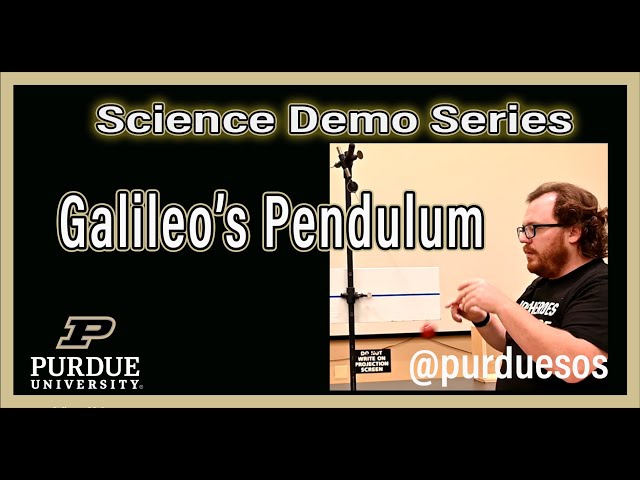The image features a slide with a solid black background and a gold-bordered rectangle in the center. Inside the gold border, the title "Science Demo Series" appears in bold white text, which is edged with black and then gold. Below this, the subtitle "Galileo's Pendulum" is prominently displayed. To the right of the text is a square photograph of a professor with glasses, a black t-shirt, red hair, and a red beard. The professor is demonstrating Galileo's Pendulum with an apparatus that includes a noticeable red ball in motion. Within the gold border, at the bottom left corner, the logo and text for Purdue University and the series title "Purdue SOS" are visible, both in white text. The overall composition effectively combines textual and visual elements to highlight the science demonstration and the affiliated institution.